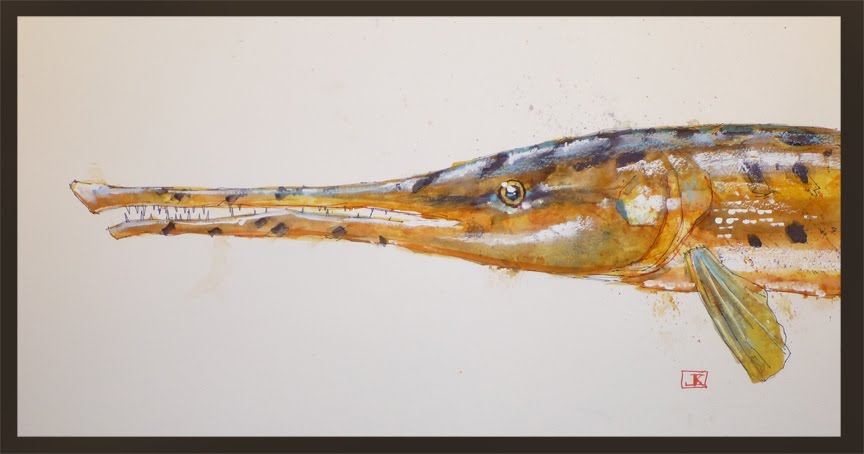The image is a detailed watercolor illustration of the front half of a gar fish, showcased on a horizontal canvas approximately two to two and a half times wider than it is tall. The fish, painted in varying shades of yellow, light orange, and brown, features numerous black spots and horizontal white stripes along its long, thin body. The artist's attention to detail highlights the fish's elongated snout filled with tiny, needle-like teeth, and its small, orangish-black eye. The background is light gray, adding to the soft, watercolor effect of the painting. Notably, the illustration is bordered by a thin black frame, enhancing its presentation. Positioned below the fish on the right-hand side is a red square bearing the initials "JK," providing a subtle signature to the artwork.